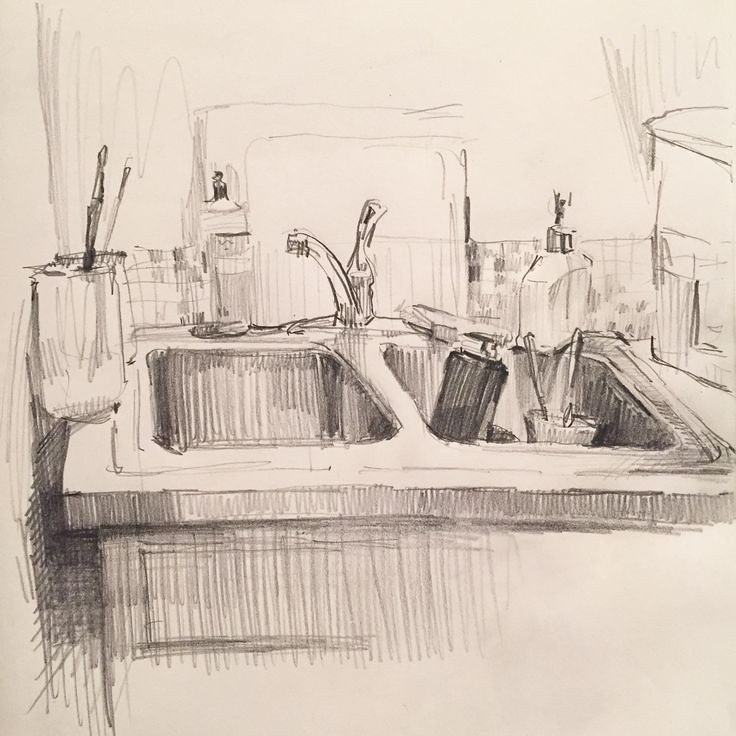This pencil sketch, done on white paper, portrays a detailed yet rough and hastily drawn kitchen scene centered around a double sink. The left sink basin is empty while the right one contains a black drink bottle and a glass with two utensil handles protruding from it. Below the sink, quick vertical and horizontal strokes suggest the under-sink structure or cabinet. 

Above the sink, on the left side against the wall, there are two jars, one placed in front of the other, each holding a paintbrush. A window is faintly sketched behind the sink, suggesting an external light source or view. Positioned between the sinks is a single-handle faucet, with a bottle featuring a push-down top, presumably for dishwashing liquid, situated to the right of the faucet. The backdrop of the scene consists of six rows of small, square tiles, adding a touch of texture and dimension to this kitchen illustration.